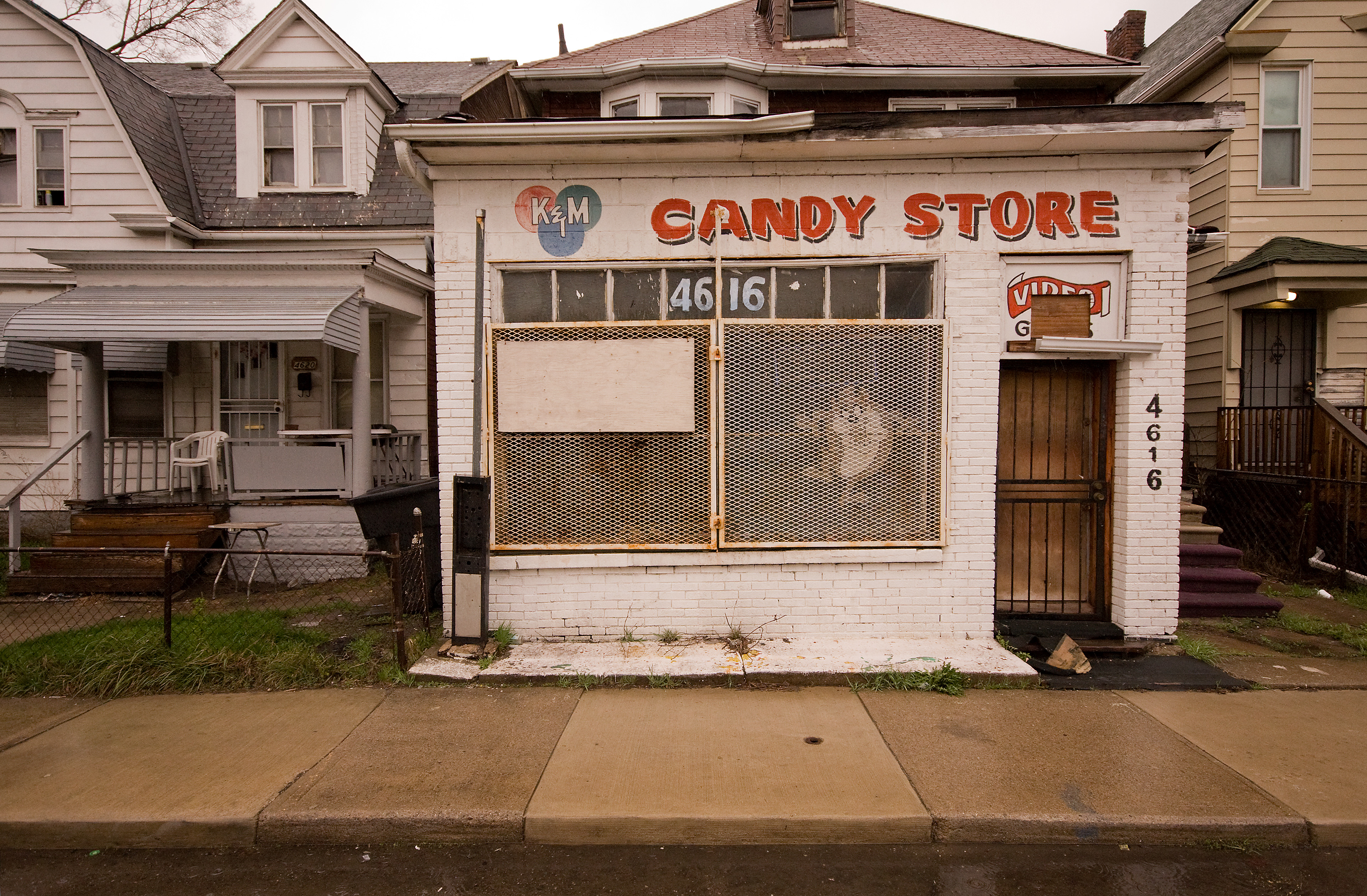This image captures a charming neighborhood scene featuring three adjoining multi-story residential houses with distinct pitched roofs, giving the setting a quaint and unified look. The houses are clearly lived in and well-maintained, adding to the authenticity of the residential area. In front of one of these houses, there stands a small, white building that contrasts strikingly with its larger neighbors — a vintage candy store named "K&M Candy Store."

The candy store, which looks as though it has weathered many years, is modest in size, comparable to a single-car garage. A nostalgic touch is added by its old-fashioned signage, with "CANDY STORE" prominently displayed in capitalized red letters. The store’s address, 4616, appears twice: once in traditional numerals on the exterior wall and vertically on the black, security-screened front door.

The façade of the candy store features two windows, both protected by sturdy grills, hinting at a time when extra security became necessary. This design choice does obscure the view inside, however. To the right of one of these windows, a smaller door boasts signage indicating the possible availability of video games, adding an extra layer of nostalgia to the setting.

The juxtaposition of the candy store against the backdrop of the residential houses is strikingly quaint. The brown sidewalk stretches across the front of the store, providing a neat and well-maintained pathway for visitors. This image perfectly encapsulates the charm of a close-knit community where unique small businesses like K&M Candy Store thrive beside residential homes.